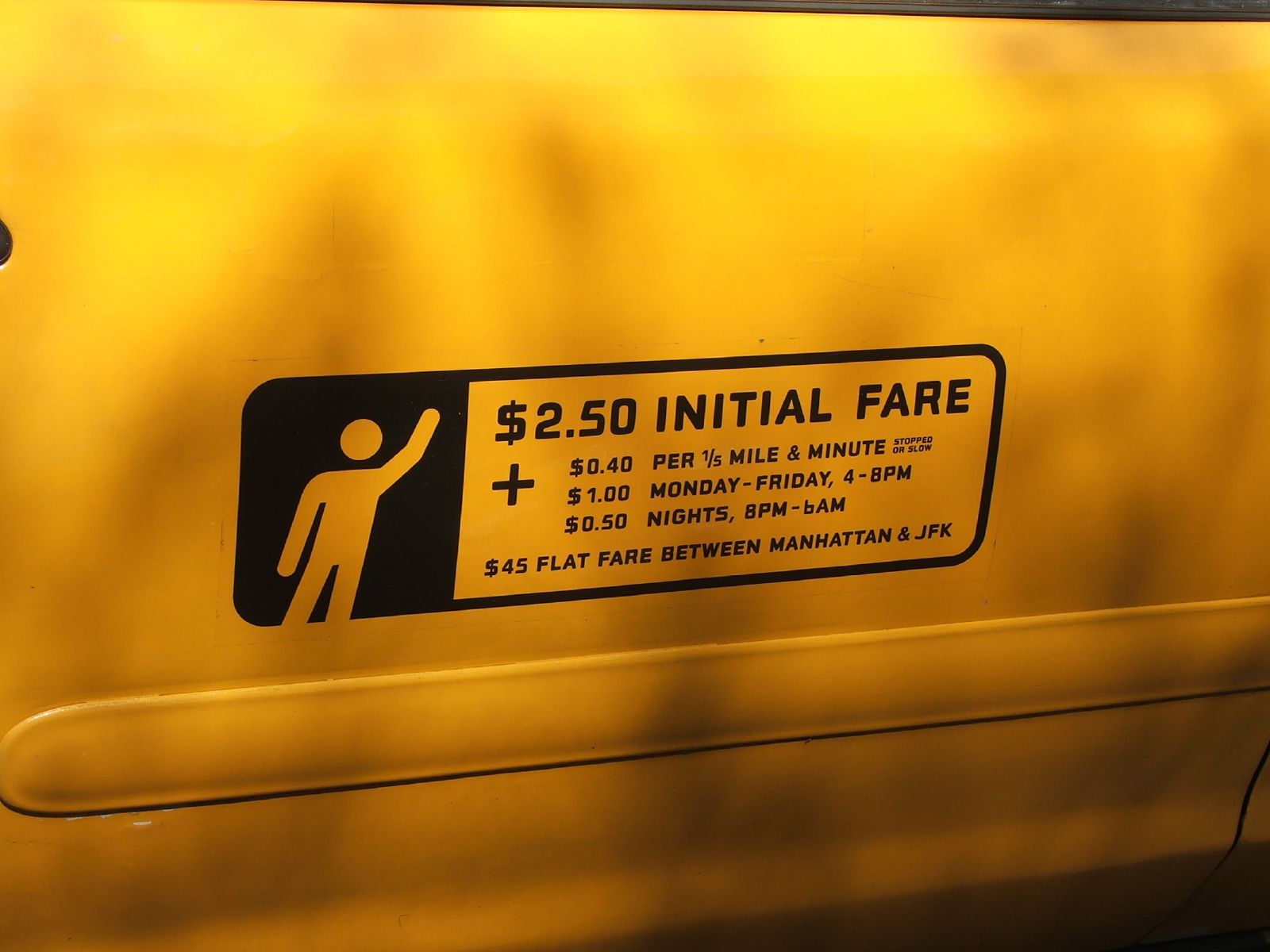This image features an informational stamp displayed on the side door of a yellow taxi cab, likely in New York City. The stamp is a black, rounded-corner rectangle contrasting with the taxi’s yellow background. Dominating the left portion of the stamp is a yellow stickman figure with one hand raised, reminiscent of a pedestrian hailing a cab. The bold black background ensures the figure stands out prominently.

Adjacent to the figure, detailed fare information is outlined in black text on varying yellow background sections. It reads:

- "$2.50 initial fare"
- "+ $0.40 per one-fifth mile and per minute, or when the taxi is stopped or moving slow"
- "+ $1 Monday through Friday, 4 PM to 8 PM"
- "+ $0.50 nights, 8 PM to 6 AM"
- "$45 flat fare between Manhattan and JFK"

This informative patch provides all necessary fare details for potential passengers and spans the entire side door of the taxi, blending seamlessly into the vehicle's design. The bottom part of the door also shows a little bit of the car’s side panel or trim, which is uniformly painted yellow to match the rest of the taxi. The image is a clear capture of a real-world fare sign, showing the specific charges and conditions for travel within the city.